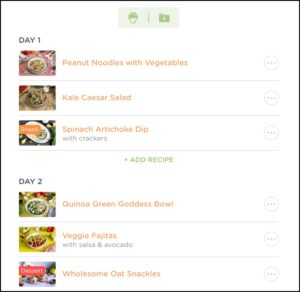The image is a vertically oriented rectangle with a white background and a thin, bold black border around its edges. At the top center, there are two light gray boxes positioned side by side, each featuring a green icon separated by a light green line.

On the left side, in bold, capitalized black font, it says "DAY ONE." Below this heading are three smaller horizontal rectangular images depicting various food items. Next to each image, on the right side in orange font, are the food descriptions. The first image is labeled "Peanut Noodles with Vegetables," the second is "Kale Caesar Salad," and the third is "Spinach Artichoke Dip." Under the third description, in black font, it says "with crackers."

Centrally located beneath these descriptions is a green plus sign followed by "ADD RECIPE" in capitalized green font.

Further down on the left side, again in bold, capitalized black font, it says "DAY TWO." This is followed by another set of three horizontal rectangular food images. Each image is accompanied by an orange font description to its right. The first food item is "Quinoa Green Goddess Bowl," followed by "Veggie Fajitas" with an additional black font note "with salsa and avocado," and the last item appears to say "Wholesome Oat Snacks," though the final word is slightly unclear.